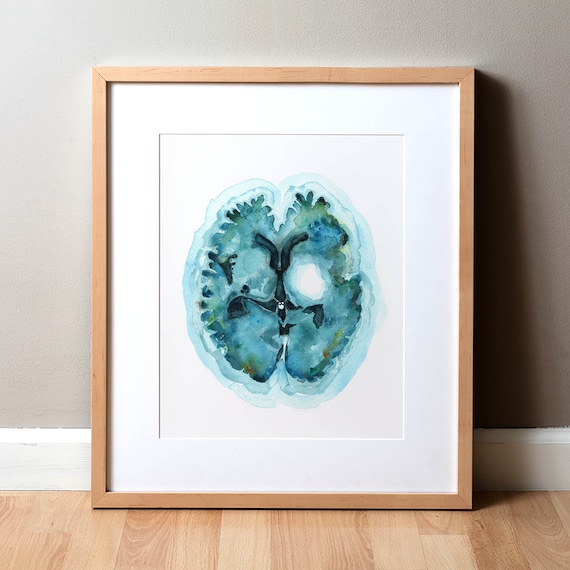The image is a detailed photograph of a contemporary watercolor painting that heavily features cooler tones such as blue and pale green, giving it an abstract and somewhat medical appearance. The painting, which is somewhat reminiscent of a Rorschach inkblot, also evokes a sense of organic forms like lungs or a cross-sectional view of the human brain. The painting's center is shaded green, with darker green accents to create depth and separation. Its edges have a fuzzy, tentacle-like texture, adding to its abstract quality.

The artwork is set against a teal or tan-colored wall, adding depth and contrasting nicely with the white matting inside its light brown wooden frame. It rests on a newly finished, light hardwood floor, contributing to a fresh and sophisticated aesthetic. The setting, likely a personal home, is modern and neat, with freshly painted white trim completing the serene and stylish environment.